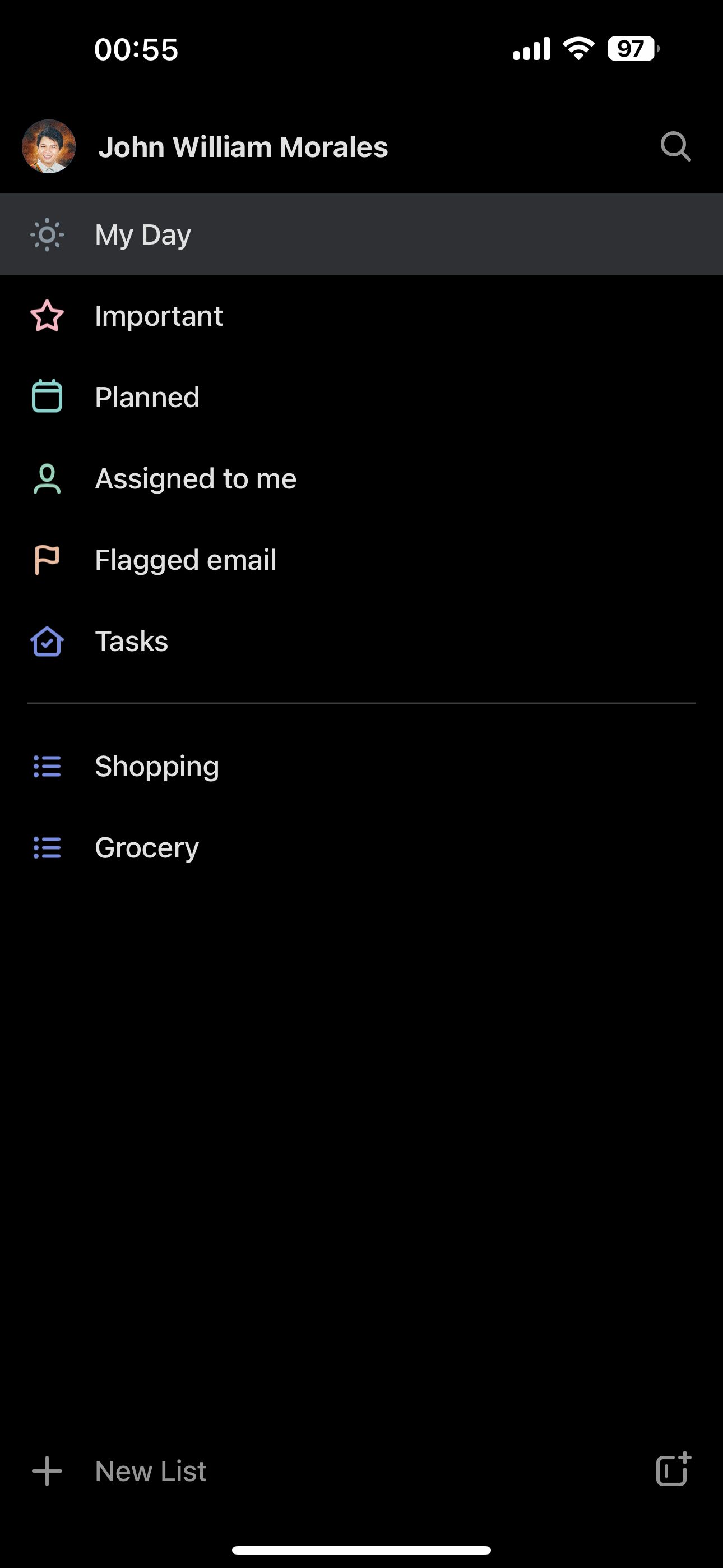This screenshot displays the interface of a tablet or phone with a predominantly black background. At the very top, the screen shows the time "00:55" in white, indicating it is five minutes to one in the morning. The device has a full cell phone signal (four bars), a full Wi-Fi signal, and a battery life of 97%. 

Beneath this top information, there is a small profile picture, though it is unclear if the person is male or female. The individual has short black hair and slightly tanned skin. The name "John William Morales" is written in white text next to the profile picture, suggesting this is likely a male. To the far right of this line is a magnifying glass icon, indicating the search function.

Below this section, the screen seems to display a planner or organizational app. It features several sections with icons and labels: a blue sun icon labeled "My Day," a pink star labeled "Important," a calendar icon labeled "Planned," an outline of a person labeled "Assigned to Me," a flag icon labeled "Flagged Email," and a purple house icon with a checkmark labeled "Tasks." 

There is a thin gray separator line followed by categories for "Shopping" and "Grocery Lists." At the bottom left of the screen, there is a plus sign with text to its right that reads "New List," indicating an option to create new lists.